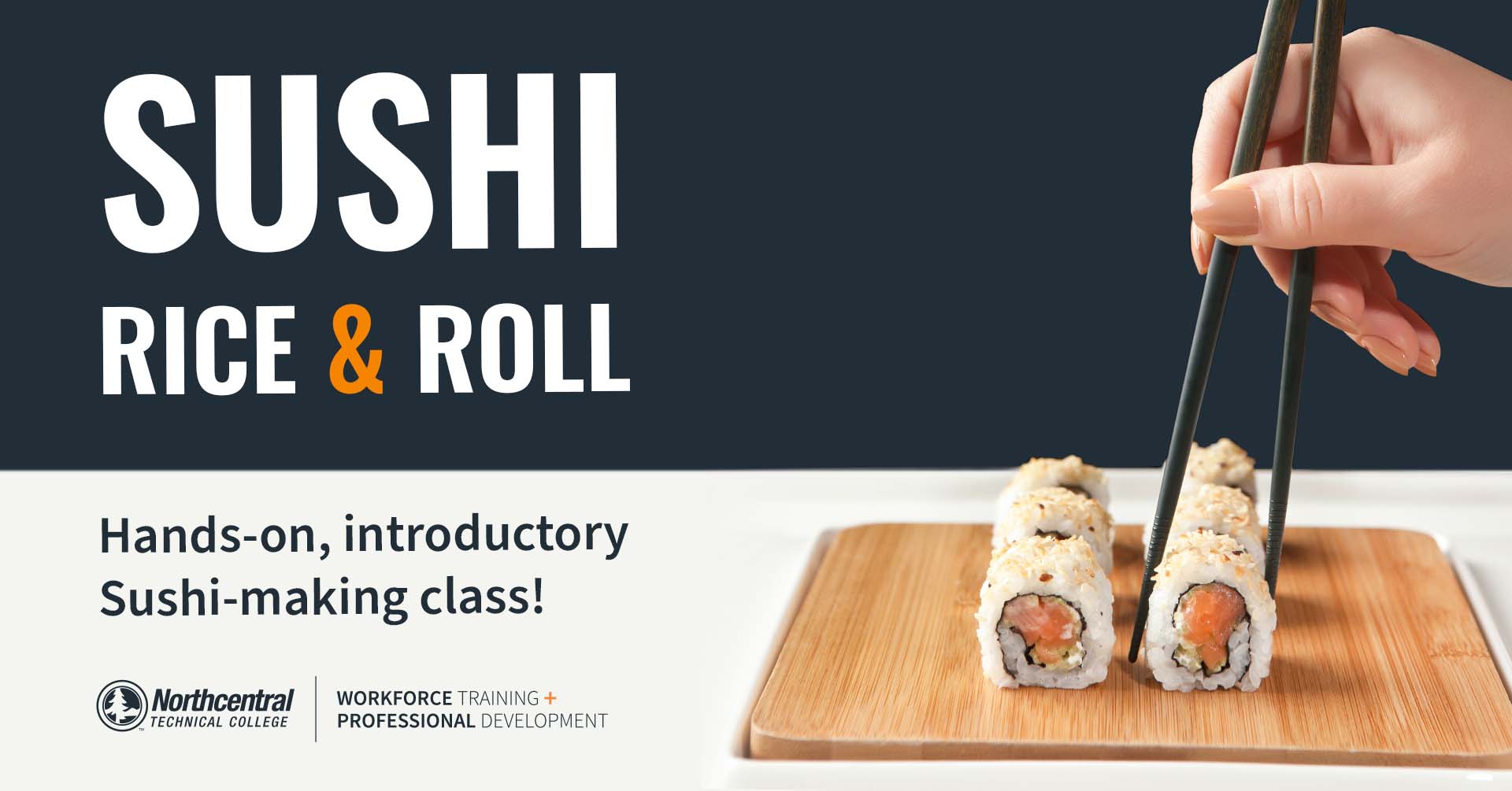The image is a detailed advertisement poster for a hands-on introductory sushi-making class at North Central Technical College, focusing on workforce training and professional development. The poster, rectangular in shape, features a prominent photograph. In the lower right portion of the image, the photograph showcases a hand of a white person with brown nail polish holding a pair of brown chopsticks, picking up a piece of sushi from a brown cutting board. The cutting board, square in shape, has a total of six pieces of sushi arranged in two rows. Each sushi piece appears to have salmon and rice, with crumbled flakes sprinkled on the outside.

On the left-hand side of the photo, there is white text that reads "Sushi Rice and Roll," indicating the nature of the class. Below it, blue text states "Hands-on Introductory Sushi Making Class," providing more specifics about the event. Towards the bottom left, the text continues with "North Central Technical College" in black, and "Workforce Training and Professional Development" beneath it. The design of the poster features a contrasting color palette: the top half has a dark blue and navy background with white and orange text, while the bottom half has a white background with black text. A small black circle with a white silhouette of a pine tree adds a distinctive logo element near the bottom left corner. The overall layout and detailed depiction aim to attract potential attendees to the college’s professional development program.